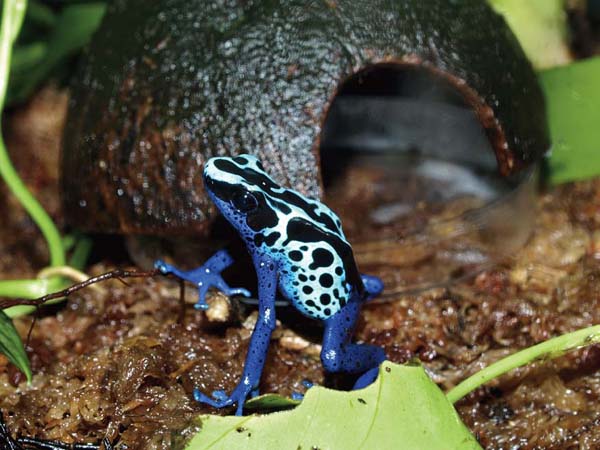In this detailed and zoomed-in image, we are presented with a vibrant and unique blue frog situated slightly above the bottom center of the frame within a terrarium. The terrarium floor is brown and slightly moist, emphasizing the natural and wet environment. The frog itself boasts a deep, radiant blue color on its legs, arms, and underbelly, transitioning to a mostly white back adorned with various black stripes and large black blotches, some resembling circles and others more oblong. The frog's head features black markings around the eyes and nose, adding to its distinctive appearance. Positioned near the frog is a large green leaf resting on the ground. Behind the frog lies a shelter that resembles a hollowed-out avocado skin or coconut shell, complete with a circular opening at the front, providing a snug refuge for the frog. To the left, there's an ascent of greenery, including vines that contribute to the lush background. The upper part of the image is dominated by green plants, enhancing the natural aesthetic of this meticulously maintained habitat.